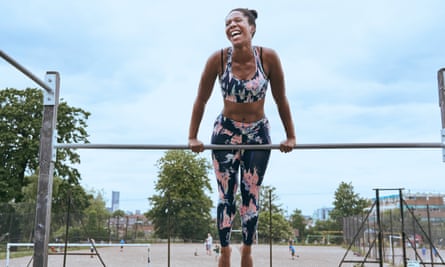In the image, an African American woman is joyfully holding herself up on a vertical bar, part of a climbing or fitness structure, in a playground or park. She is clad in a matching blue and pink tie-dye sports bra and capris covered in large floral patterns. Her dark hair is pulled back into a bun, and with her arms extended straight and wrapped around the bar, she faces the camera with a head tilt to the left, exuding happiness. The setting appears urban with a blend of natural and man-made elements; there are trees, a volleyball net, fencing, and faint outlines of buildings and large structures against a partly cloudy sky. The background is dotted with indistinguishable people engaging in various activities, adding to the vibrant atmosphere of the fitness-focused park.